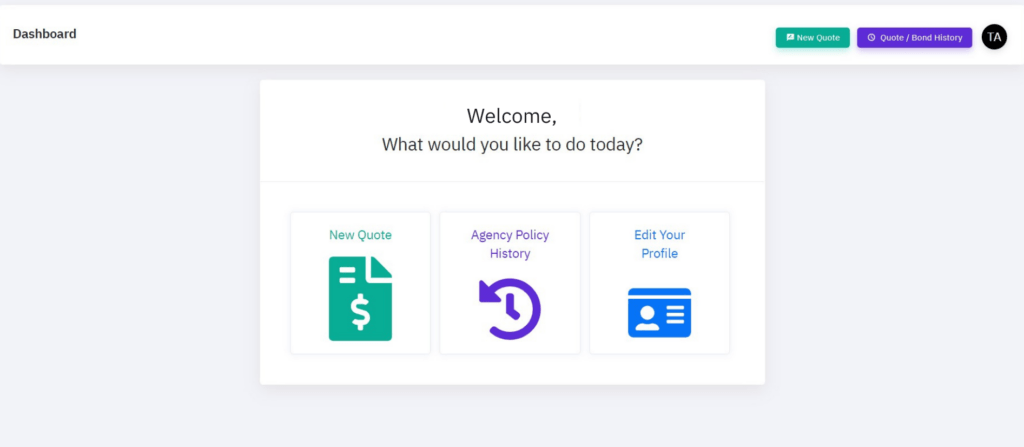The image depicts a user dashboard page from an insurance agency. In the upper left corner, the word "Dashboard" is printed in black. To the upper right, there is a green box labeled "New Quote," followed by a blue rectangular box that reads "Quote/Bond History." In the far upper right, a black circle with white text features the initials "TA."

The banner beneath this section is gray, spanning the page, with a centrally-located white rectangle containing text and several logos. The text at the top of this rectangle, centered in black print, reads "Welcome, what would you like to do today?" Beneath this greeting, three squares are arranged horizontally, each with a unique icon and accompanying text.

The leftmost square displays an icon of a piece of paper with a folded top right corner and a dollar sign in the center. Above the paper, the text reads "New Quote." The middle square features an icon resembling a partial circle with an arrow and clock hands, labeled "Agency Policy History." The square on the far right shows an icon that looks like a driver's license with a profile of a person and several horizontal bars, topped by the text "Edit Your Profile."